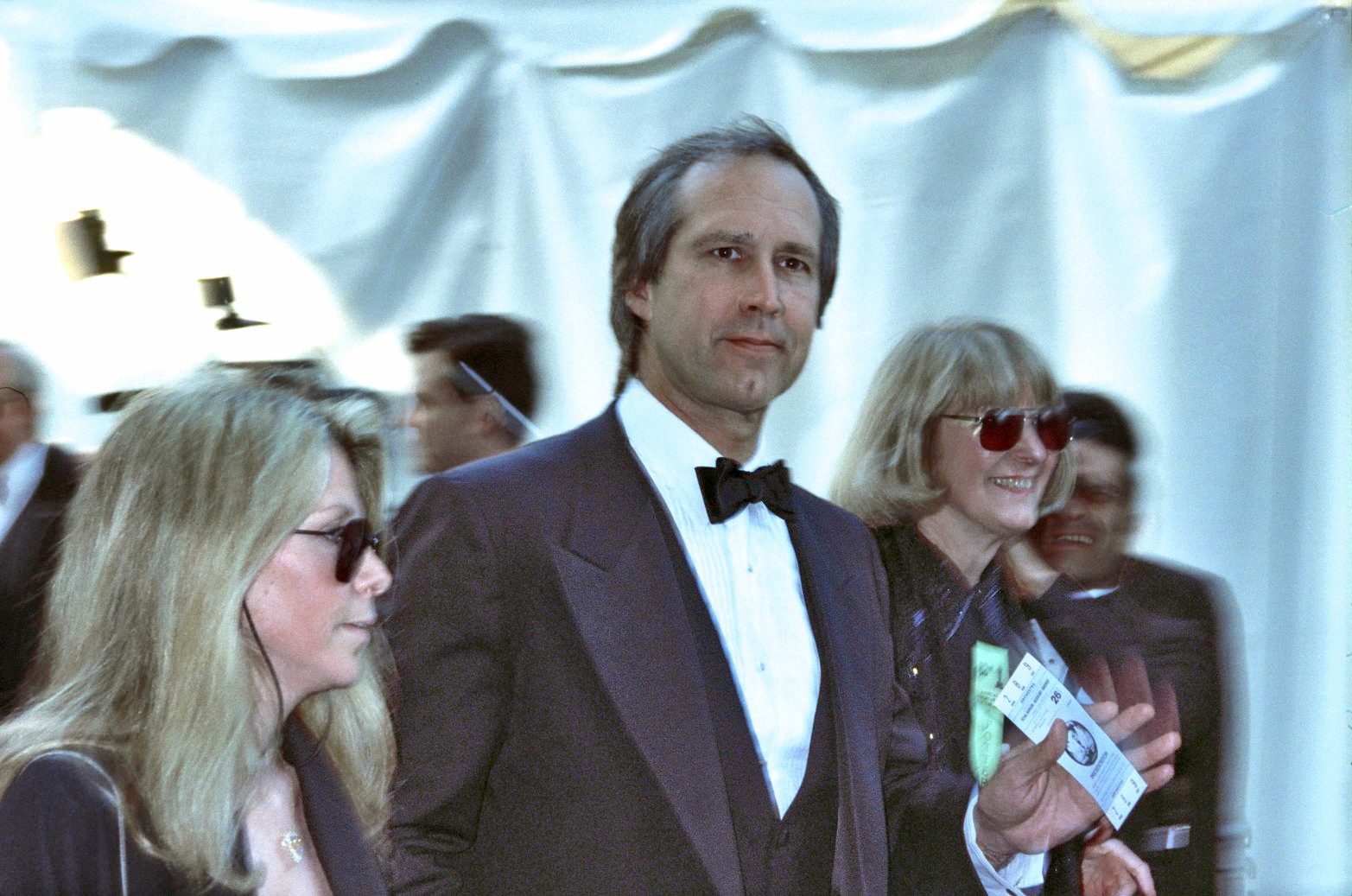The image is a color photograph in landscape orientation featuring the renowned actor Chevy Chase, likely taken in the late 1980s. Chevy Chase, with a partially receding hairline and nicely combed hair, is dressed in a black tuxedo complete with a white shirt, black satin lapels, and a black bow tie. He appears to be looking slightly to the upper right, holding what looks like a ticket stub in his left hand.

Flanking Chevy Chase are two women with blonde hair, both wearing dark sunglasses. The woman on his left, closer to the camera, has longer blonde hair cascading past her shoulders. She is dressed in a blue v-neck outfit and sports a gold necklace, with a purse slung over her shoulder. The other woman, to his right, has short, chin-length blonde hair and is wearing a black collared shirt.

The trio stands against a backdrop of a white curtain with scalloped details at the top. Other people can be seen in the background but are blurry, including a man who appears to be holding a camera over his shoulder, partially obscured by one of the women. The photograph's style is rooted in representational realism, capturing a candid moment from an event many years ago.